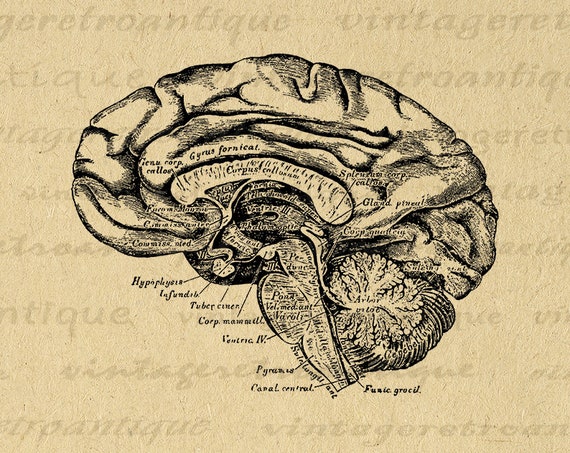The image is a detailed black and white drawing of a human brain, meticulously labeled to highlight its various sections and components. The brain illustration is overlaid on a background of semi-transparent printed words, giving it a vintage, retro feel. The labels on the brain include terms such as hypothalamus and hypophysis, among others, with arrows and lines pointing to the specific parts. The diagram is clean and precise, capturing the intricate details and slight curvature of the brain. The numerous labels and terms are scientific in nature, reflecting a thorough and educational approach to the depiction.